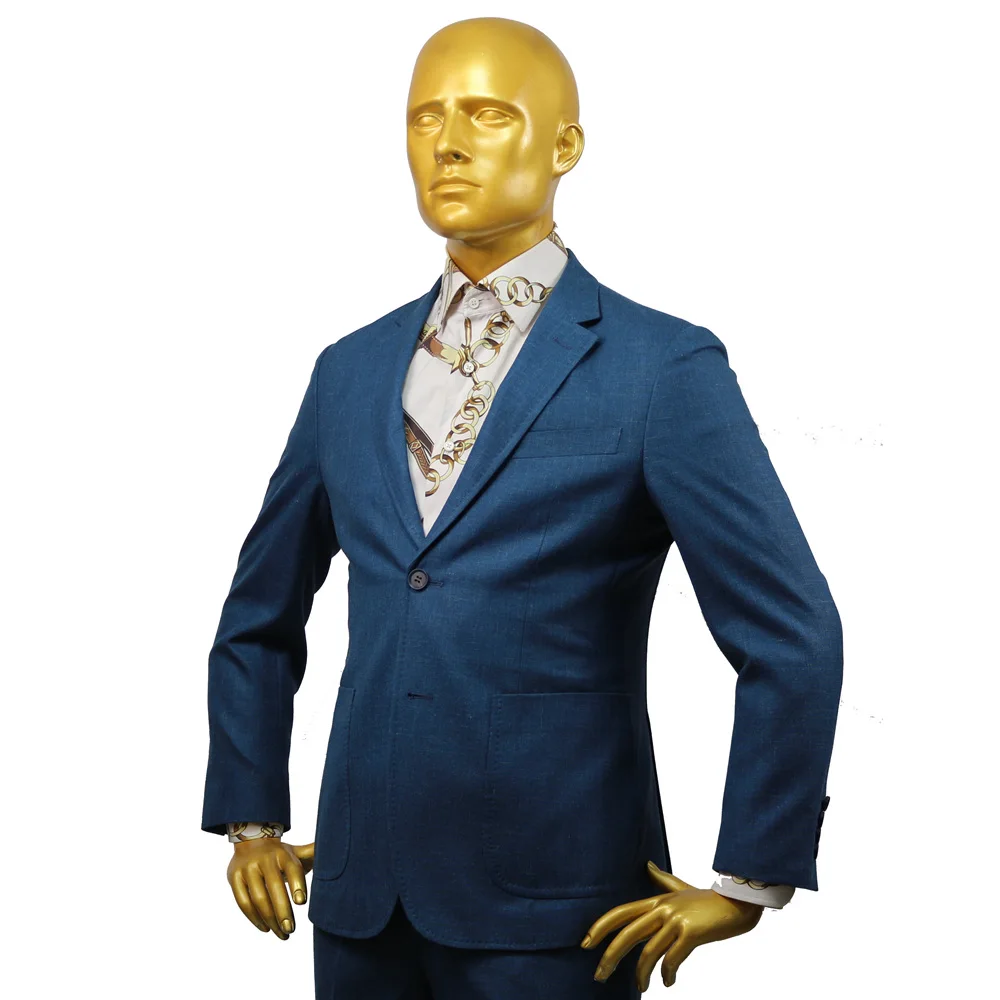This is a photograph featuring a glossy, gold-colored mannequin with a bald head and featureless, gold eyes. The mannequin is garbed in a vibrant dark blue suit consisting of a single-breasted jacket—buttoned once below the breastbone—and matching blue trousers. Underneath the jacket, the mannequin sports a long-sleeve, off-white button-up shirt adorned with intricate, gold-patterned decorations resembling chains or circles that extend to the cuffs. The mannequin stands in a confident pose with hands on hips and shoulders back, exuding a somber expression while gazing to the left. The white background and frontal lighting suggest that the image is intended for an online store or catalog to showcase the suit comprehensively.